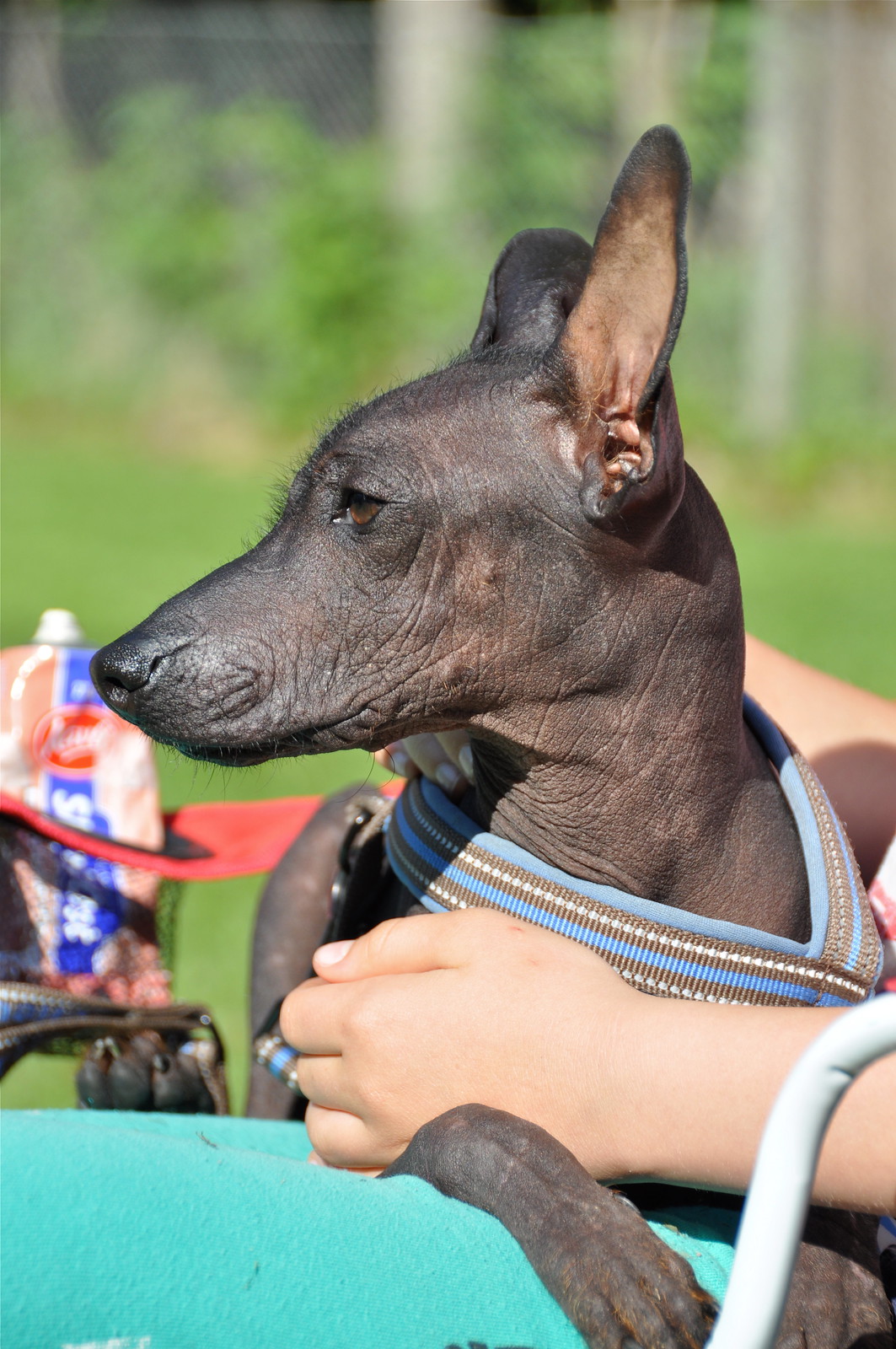This is a detailed close-up photograph of a hairless dog with a dark gray, almost black, skin tone, taken outdoors during the day. The dog features long, tapering ears with brown inner parts and a distinctive, elongated snout, visible in profile as it faces to the left. Its paws rest on a light blue object that appears to be a bench. The dog is adorned with a thick collar or harness featuring multiple layers of blue and brown stripes with white dots. A pair of white hands gently holds the dog, providing a sense of scale and connection. The background is softly blurred, featuring indistinct trees and leaves, contributing to a serene outdoor setting. In the lower right-hand corner of the image, a handle is partially visible, and a package with unreadable text is also out of focus behind the dog's nose.